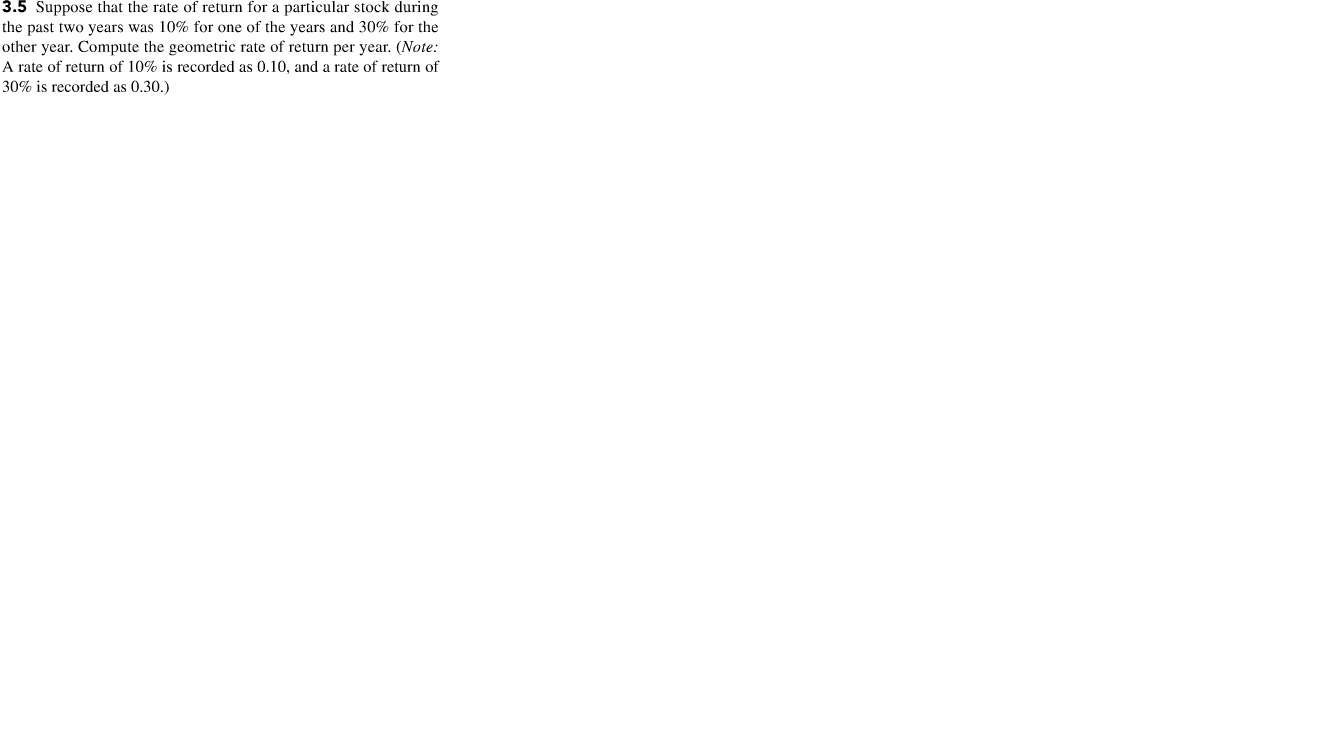This image focuses on an exercise labeled "3.5" in the upper left corner, which presents a mathematical problem related to the geometric rate of return for a particular stock over two years. The text on the image is quite small and difficult to read, and it's displayed in black against a stark white background.

The exercise states that the stock had a rate of return of 10% for one of the years and 30% for the other year. It instructs the reader to compute the geometric rate of return per year, noting that a 10% return is recorded as 0.10 and a 30% return is recorded as 0.30.

Other than this concise mathematical problem, the image is entirely blank, and there are no additional indicators as to its origin, such as whether it's a page from a textbook or a screenshot from another source.